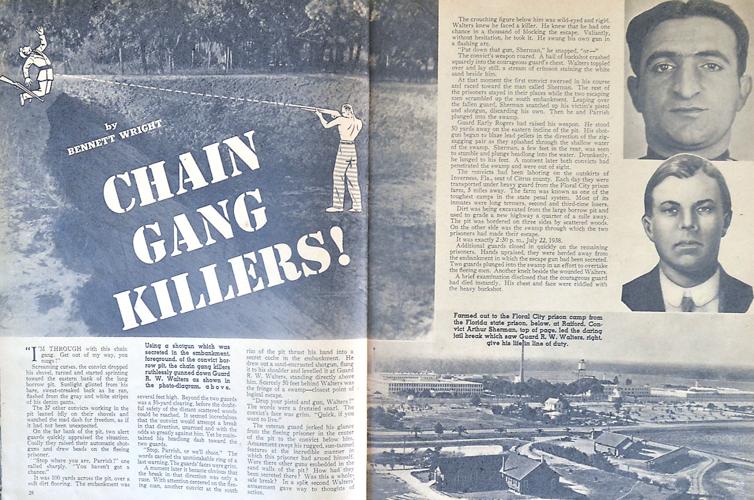This image is a scan of a vintage magazine article, likely over 50 years old. The focal point of the scan is the fold indentation down the center, characteristic of an opened magazine or pamphlet. The article, featuring several paragraphs of black text on a white background, is interspersed with stylized images and illustrations. 

Prominently on the left side of the article is a large black and white photo of an outdoor setting, superimposed with a cartoon-like drawing of two men: one man is shooting a rifle while wearing striped pants, aiming at another man who is an officer falling forward. This image is captioned "Chain Gang Killers! by Bennett Wright." 

On the right side of the article, there are two black and white headshots of two different men. Both men have white skin, with dark hair that is side-parted, bushy eyebrows, wide-set eyes, large noses, and thin lips. Below these headshots is another black and white photo depicting an aerial view of a city or town, showing various buildings, roadways, trees, and bushes. The article comprises multiple columns of text, primarily in black and white, with quotes and detailed captions enhancing the narrative.